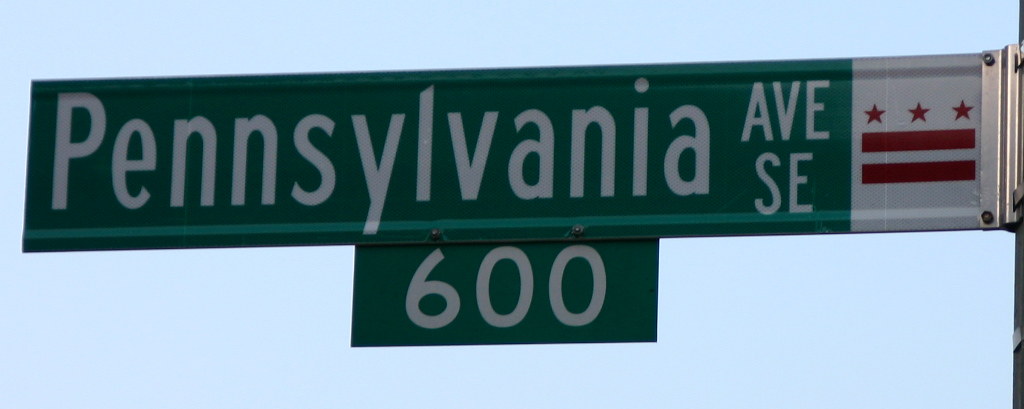This is a detailed and clean caption for the image:

"A close-up photograph of a street sign for 600 Pennsylvania Avenue Southeast, likely in Washington, D.C. The dark green street sign features 'Pennsylvania Avenue SE' in bold white letters, with '600' displayed directly below it. To the right of the street sign is a white partition adorned with three red stars above two red bars, a design reminiscent of the D.C. flag. The sign is set against a clear, light blue sky, and a small part of the pole supporting the sign is visible on the right-hand side of the image. The focus on the street sign against an uncluttered sky provides a crisp and clear representation of this notable address."